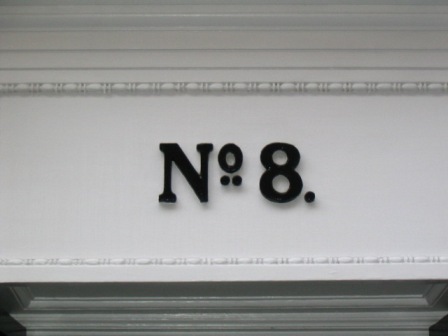The image features the house number "No. 8" displayed in black lettering on a white wall. The "N" is capitalized, and the "O" is small with two black dots centered beneath it. There is a period following the number 8. The white wall seems to be part of a column, mostly extending out of the frame at the bottom, with a black background behind it. At the top and bottom of the wall, there are white ridges, with a prominent, decorated white lip at the very top. The setting of this display suggests it is situated above a doorway or on the lintel of a door, possibly part of the ornate exterior of a building featuring intricate wood trim and carved inlays.